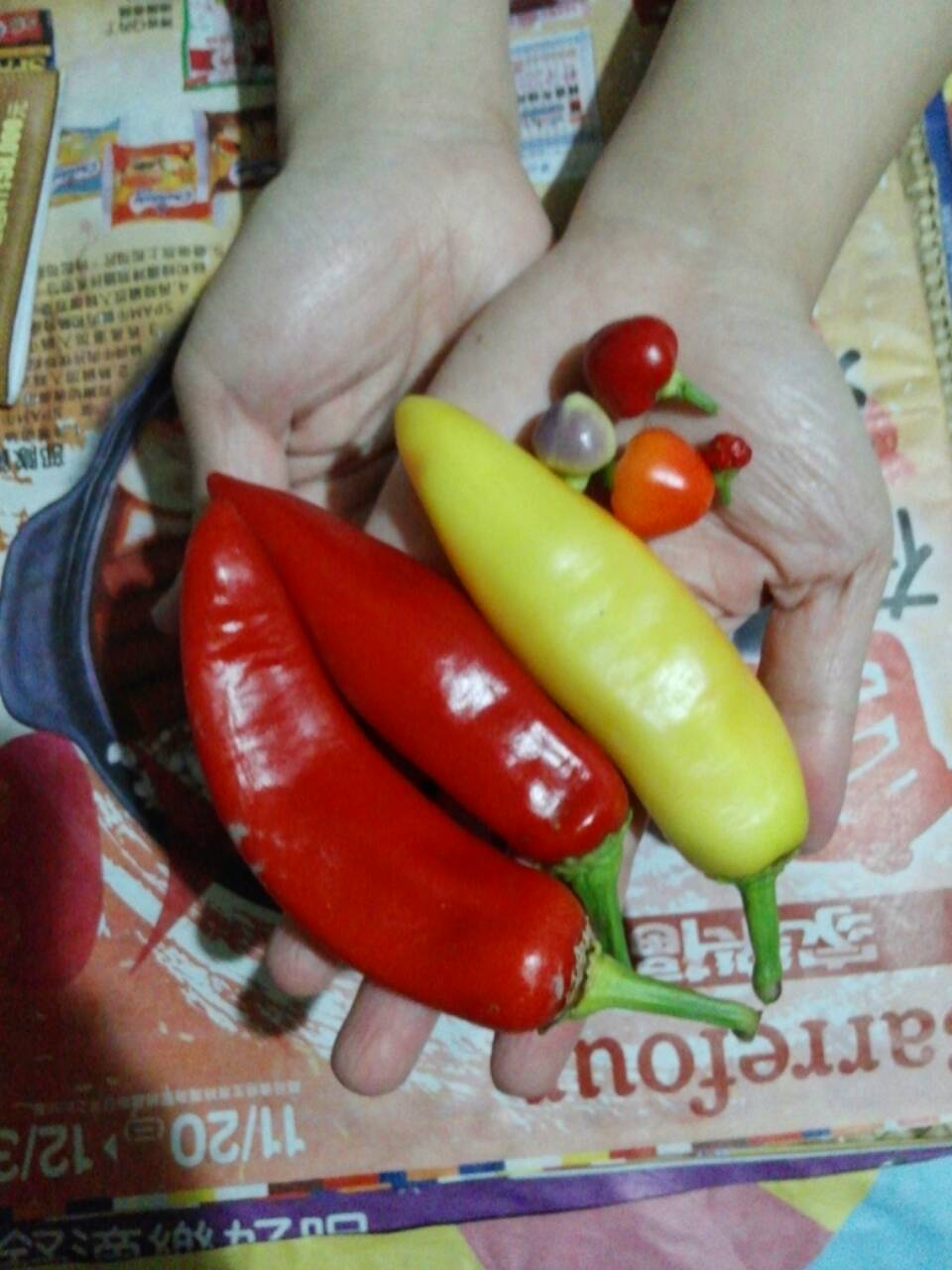This is a color photograph taken indoors, capturing a pair of white hands holding an assortment of peppers. The hands, shown from just below the wrists to the fingertips, come together in a V-shape in the center of the image, palms facing up. In the hands are two long red peppers and one long yellow pepper, all with green stems. Additionally, there are tiny, round, peculiarly shaped red and orange peppers, resembling stones. The background beneath the hands is a colorful newspaper, printed with Japanese characters and featuring various vibrant hues of red, white, and yellow.